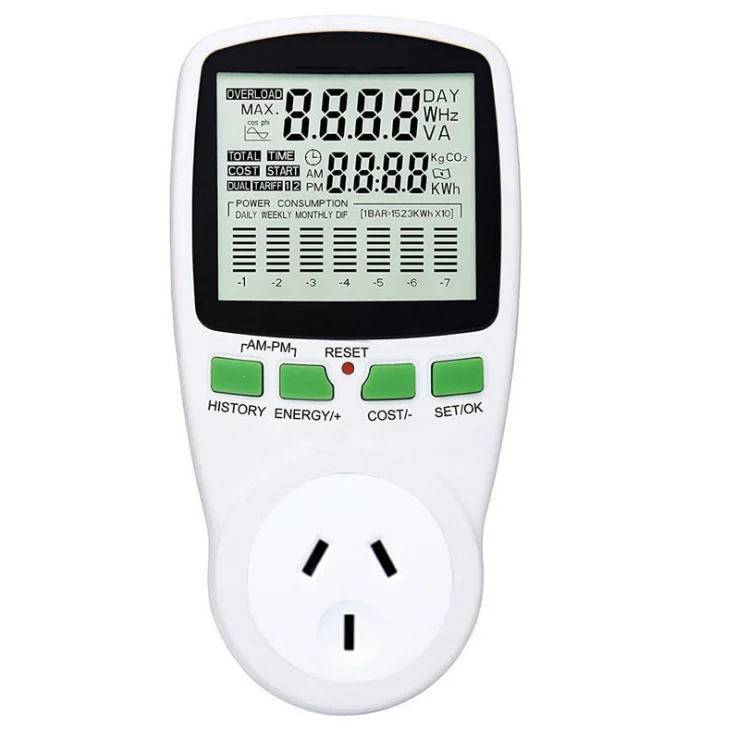The image showcases a digital monitoring device predominantly made of white plastic, set against an all-white background. Central to the device is a gray screen displaying various placeholders and symbols such as '8888', 'W-H', 'G-B', 'A', 'C', 'G-C-O-2', a dollar sign, 'K-W-H', 'Max', 'Total time', 'cost', 'start', 'call', 'tariff', 'AM', 'PM', and 'Power consumption daily, weekly, monthly'. The text on the screen are in black, outlined by a black frame. Below the screen, there are four green buttons labeled 'History', 'Energy/Plus', 'Cost/Minus', and 'Set/OK'. At the center of these buttons is a small red 'Reset' button. Additionally, there are three black plug-like slots at the bottom of the device. The device appears well-marked with descriptors and functional symbols, emphasizing its role in monitoring and displaying detailed electrical or energy-related information.